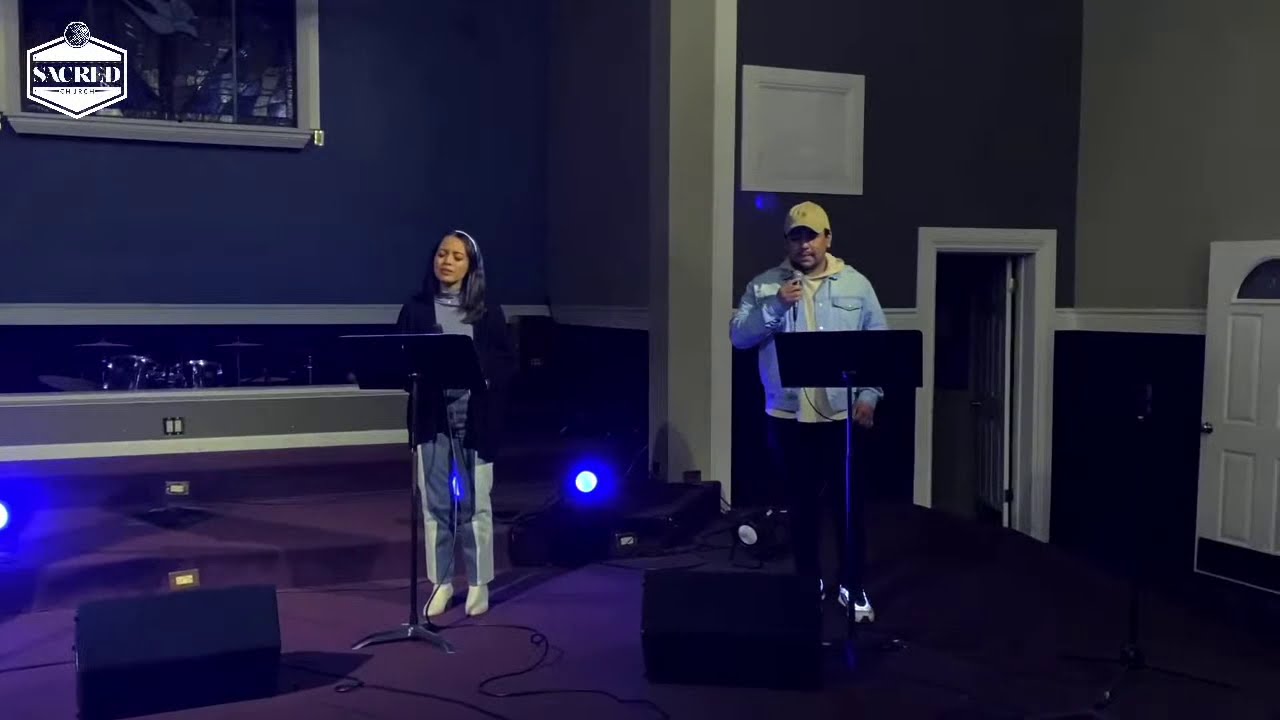The image depicts a man and a woman standing on a stage, likely in a church, preparing to perform a duet. The stage features a rich purple carpet and dark navy blue walls, accented by blue lights near the floor. Both individuals are positioned behind black music stands.

The woman, situated to the left, has long brown hair and wears a black cardigan over a blue shirt, light blue jeans with white stripes down the sides, and white shoes. She appears absorbed in the moment, possibly singing. To her left and slightly below her, a bright blue light is visible, casting an aura.

To the right, the man wears a light blue denim jacket layered over a yellow hoodie, black pants, white sneakers, and a tan khaki hat. He holds a microphone close to his mouth, indicating he is speaking or singing. Behind him, a white-trimmed doorway is visible, emphasizing that the stage is elevated.

The background includes another door and possibly a large window, contributing to the room's church-like ambiance.